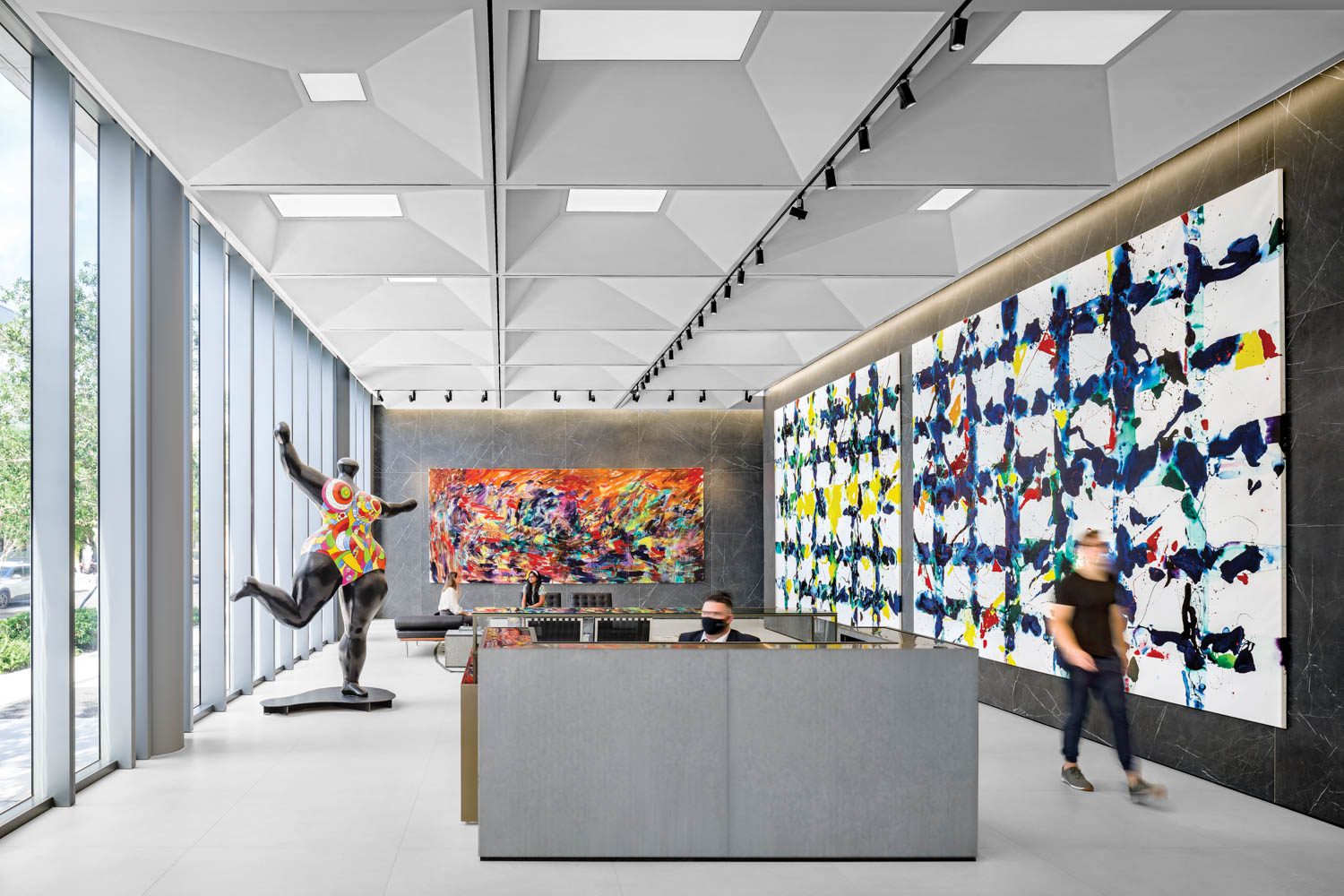This image captures the interior of an art gallery. To the left, floor-to-ceiling windows allow natural light to flood the space. Adjacent to these windows is a striking mural composed of bright, block-like colors that dominates the entire left wall. At the back of the room, another large mural features an array of colorful, splashy, modern art. The left side of the room also showcases a sculpture of a heavyset woman adorned in a vividly painted one-piece bathing suit, standing on one leg with arms and the other leg outstretched. Central to the room is a high desk, behind which a man, seated low and wearing a black mask, attends the gallery. Another individual, also masked, walks along the right side of the room, seemingly inspecting the artwork. The environment suggests a setting contemporaneous with the COVID-19 pandemic.